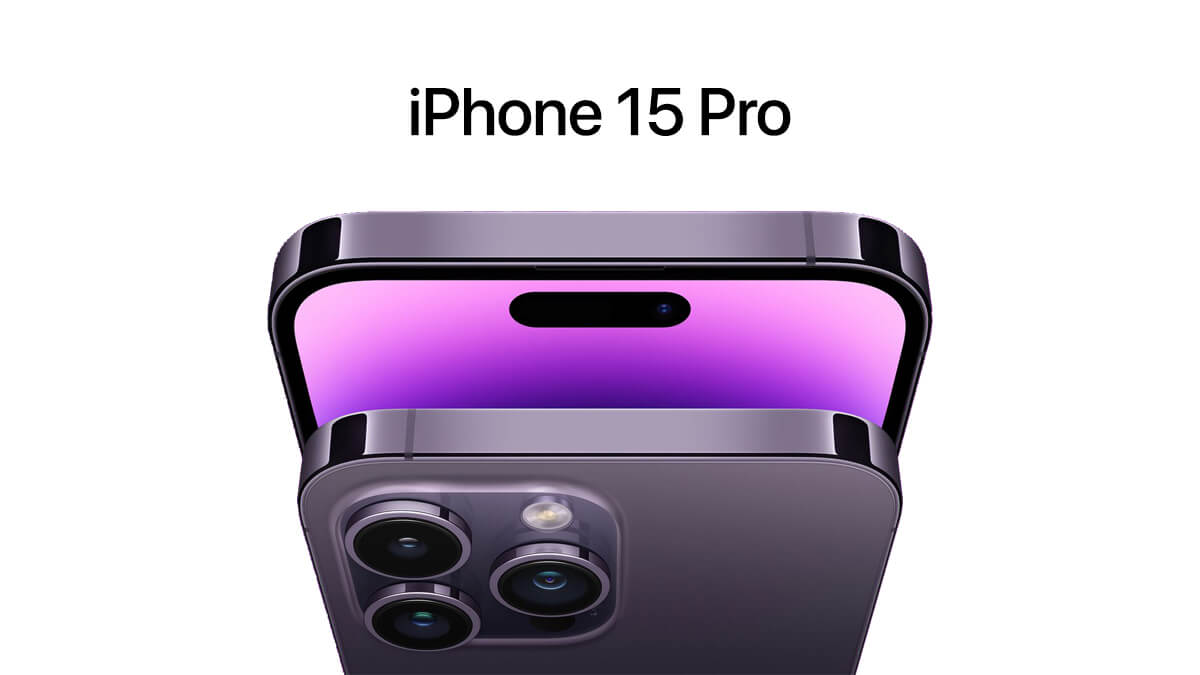This photograph showcases two iPhones, one captured from the back and the other from the front, positioned closely together as viewed from above. The devices feature a sleek, silvery-purple finish on their metal backs and edges. The rear of the phone prominently displays three camera lenses encased within a raised, square area with rounded corners, alongside a silver and white flash component.

The front screen exhibits a gradient of colors ranging from dark purple to lighter purple and pink, bordered by a black bar at the top and shiny metallic edges. Above the phones, the text "iPhone 15 Pro" is displayed in black against a white background. The bottom portion of both phones is cut off just below the camera area.

The camera lenses reflect hues of blue and green, adding a dynamic touch to the overall appearance. The image is centrally composed with a white background, highlighting the vivid metallic and gradient color scheme of the devices.